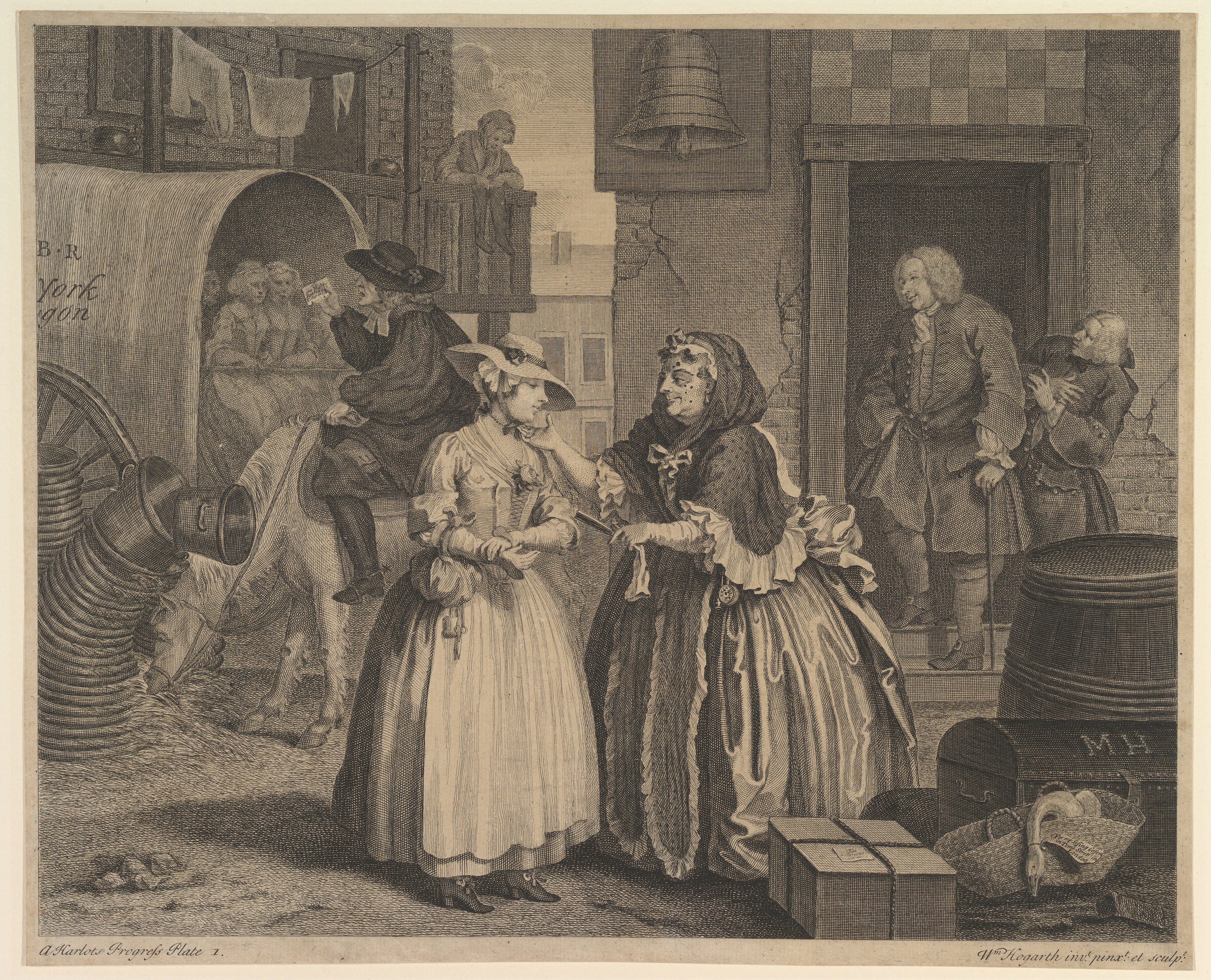This detailed, black-and-white illustration, titled "A Harlot's Progress: Plate One" by H. Hogarth, is an old engraving from the 1700s, rendered on a lightly weathered beige canvas. The image is a bustling street scene outside a deteriorating brick building with a wooden balcony. In the foreground, an older woman, dressed in an extravagant, puffy dress with a shawl hood over her head, gently holds the chin of a younger woman to her left, who is adorned in a large dress and a flower-adorned straw hat. The younger woman also carries a bag on her arm. The street is littered with suitcases and wooden boxes. In the background, two men with powdered wigs stand in a doorway; one holds a cane. Additionally, a man on horseback engages with women inside a covered wagon. Overlooking the scene, a woman stands on the balcony, seemingly drying clothes. A large bell hangs next to the doorway where the men are positioned. The overall atmosphere is dark and dreary, with intricate details capturing the lifelike quality of this 18th-century setting. Fine cursive text in the corners adds to the historical authenticity of the illustration.